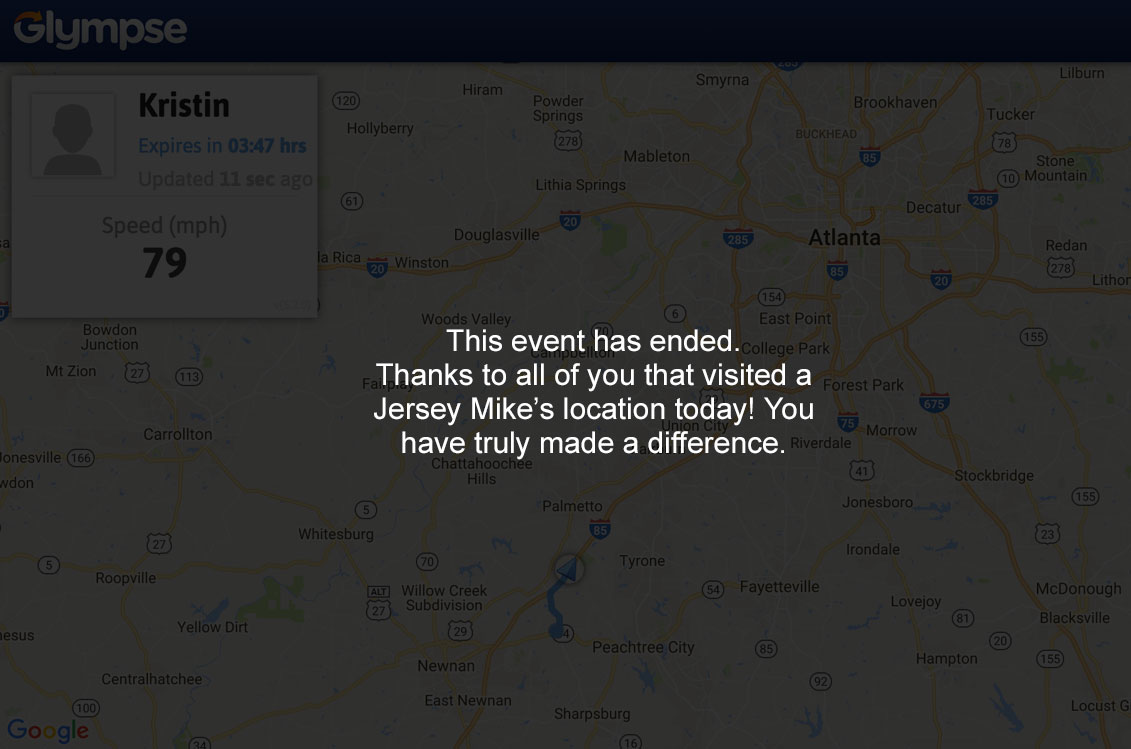The image features a black background with a faintly visible map in the backdrop highlighting cities such as Peachtree City, Fayetteville, Tyrone, Willow Creek, Whitesburg, and Atlanta. Prominently, there is a white box displaying a profile image and text indicating "Kristen" with additional details including the event expiration time of 3.47 hours, an update from 13 seconds ago, and a speed of 79. In bold, white text across the front, it announces, "This event has ended. Thanks to all of you that visited at Jersey Mike's location today. You have truly made a difference." The word "glimpse" is also printed in white text partially visible behind the foreground elements, providing a central focus to the composition.